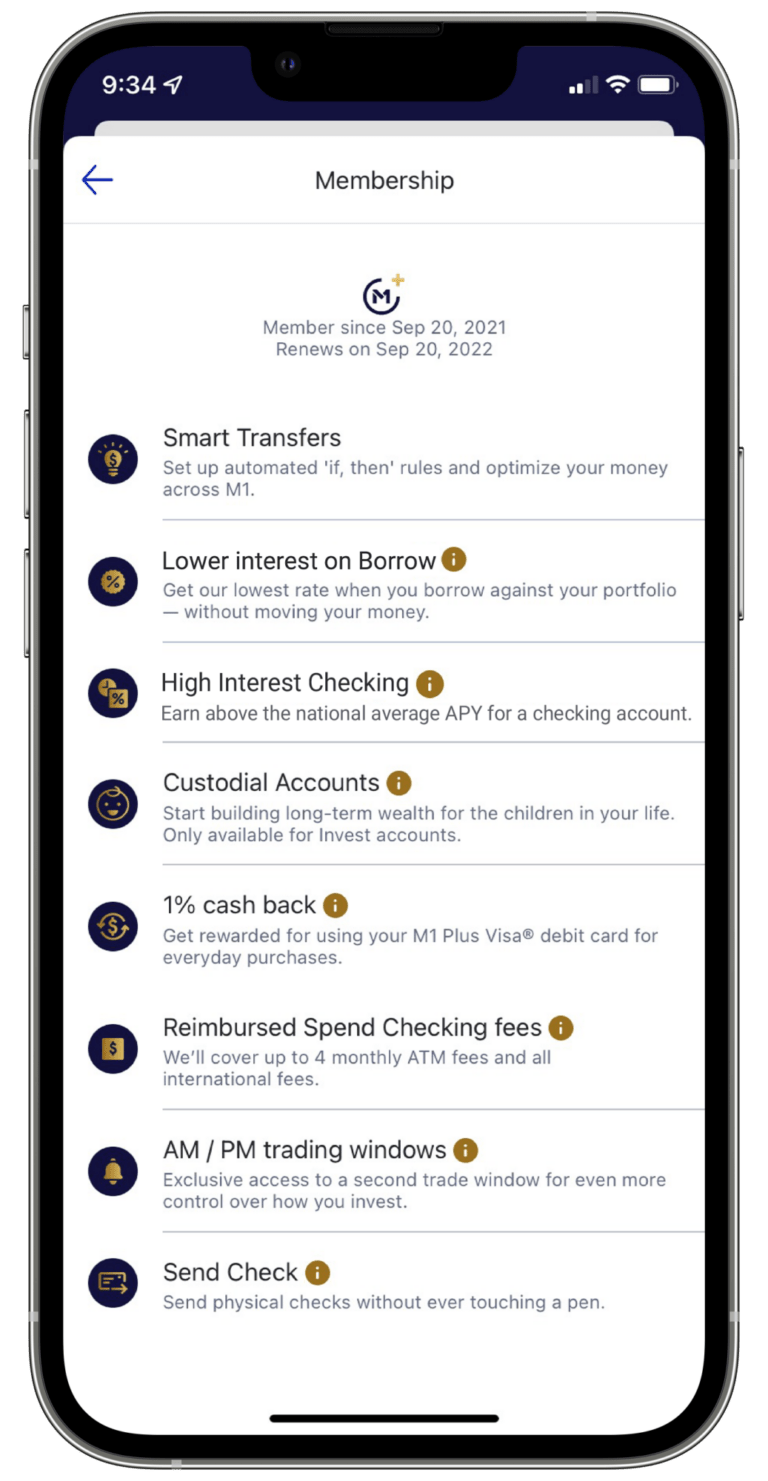This image showcases a cell phone displaying the screen of a financial management app at 9:34 AM. At the top of the screen, it prominently indicates the user's membership status: "Members since September 20th, 2021. Renews on September 20th, 2022." The screen includes a variety of features and benefits offered to the user.

A highlighted section features a light bulb icon, denoting "Smart Transfers." It promotes setting up automated If-Then rules to optimize money management across the M1 platform.

Further down, an advertisement illustrated with a percentage sign emphasizes "Lower Interest on Borrow," encouraging users to borrow against their portfolio at the lowest available rate without moving their funds.

The next section highlights "High Interest Checking," advertising above-average national APY rates for a checking account.

Additionally, the app offers "Custodial Accounts," inviting users to start building long-term wealth for the children in their lives—note that this option is only available for invest accounts.

A "1% Cash Back" feature is also promoted, rewarding users for everyday purchases made with the M1 Plus Visa debit card.

Lastly, the screen mentions the benefit of "Reimburse Spend Checking Fees," offering to cover up to four monthly ATM fees and all international fees.